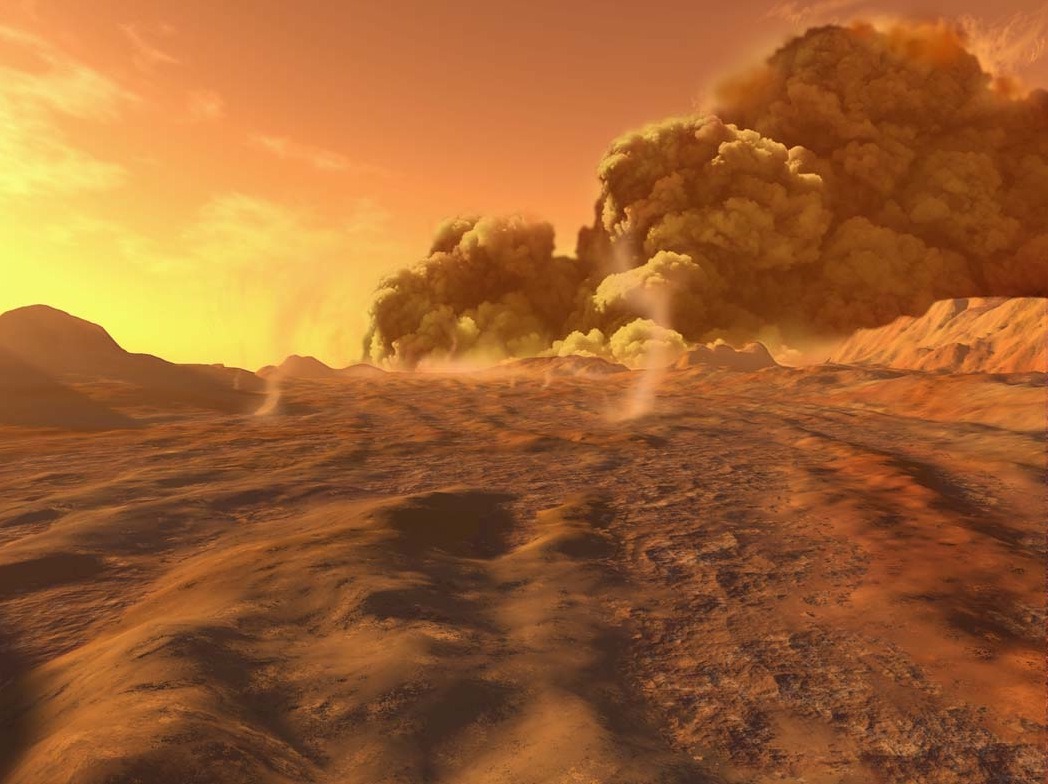The image depicts a barren, desert-like landscape with dry, cracked ground and craggy rocks in the background, reminiscent of Mars. The scene is dominated by a massive column of brown-yellow smoke billowing upwards, likely from a volcanic eruption. The smoke is rising from the earth, suggesting recent volcanic activity, and is blown towards the right by the wind. There is no vegetation visible, enhancing the desolate feel of the area. The sky is imbued with dark, dramatic hues ranging from yellow to deep red, possibly intensified by the smoke. Despite the apparent devastation, the image is bright and clear, with the lighting emphasizing the reddish, rusty color of the earth. The horizon shows a glow that could be from a rising or setting sun, adding to the dramatic effect. The overall tone of the image is strikingly orange, mirroring the intense heat and activity at the scene.